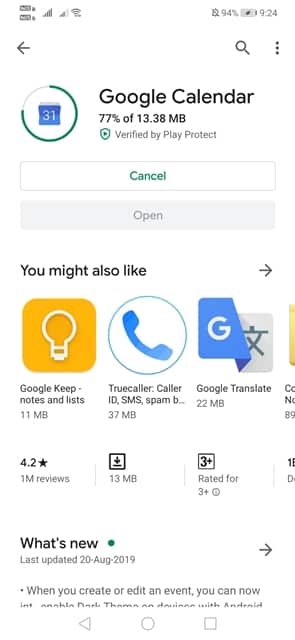**Detailed Caption:**

The image is a screenshot from the Google Play Store on what appears to be a smartphone. At the very top, the status bar displays a couple of notifications, likely from Google Meet, along with icons for Wi-Fi and a battery indicator showing 94% with the device currently charging. The current time shown is 9:24.

Below the status bar, the main interface of the Google Play Store is visible. The layout includes a left-facing arrow for navigation, a search magnifying glass, and a hamburger menu icon. Directly beneath these icons, a section displays the Google Calendar app in the process of downloading, with a progress bar showing 77% completion (13.38 megabytes downloaded). The circular progress indicator features the number "31."

The app is marked as verified by Google Play, and users have the option to cancel the download or open the app once it's fully installed (the "open" button is grayed out until installation is complete).

Further down, there's a section titled "You Might Also Like," accompanied by a right-facing arrow to scroll through recommendations. The first few suggested apps are shown with matching icons: Google Keep, Truecaller, and Google Translate.

Below the suggestions, additional details include the app's size and user reviews, along with a section titled "What's New" marked by a green dot. This section provides a brief, truncated summary of the latest updates to the Google Calendar app, including the last update date. The description cuts off, not showing the entire update information.